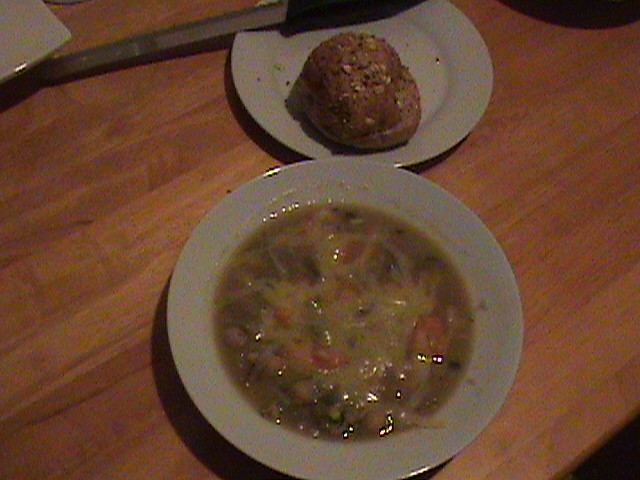This color photo captures a close-up view of a hearty meal set on a light brown tabletop. Central to the image is a bowl of soup, positioned towards the bottom two-thirds of the composition. The soup has a rich, brothy base, transitioning from yellow at its core to a muddied brown at its edges. Within the soup, there are visible pieces of carrot and hints of other vegetables, possibly complemented by noodles. The soup is topped with what looks like melted cheese, adding a creamy layer to the dish.

Behind the bowl, a white ceramic plate holds a whole grain roll, its brown crust adorned with various seeds and grains, possibly oats. This bread roll adds a rustic touch to the presentation. To the right side of the image, slightly cropped, is a utensil with a black handle and a silver blade, likely a serving spoon or a pair of tongs. The top left corner of the image shows the edge of another ceramic dish or plate, adding to the cozy, homely feel of the scene.